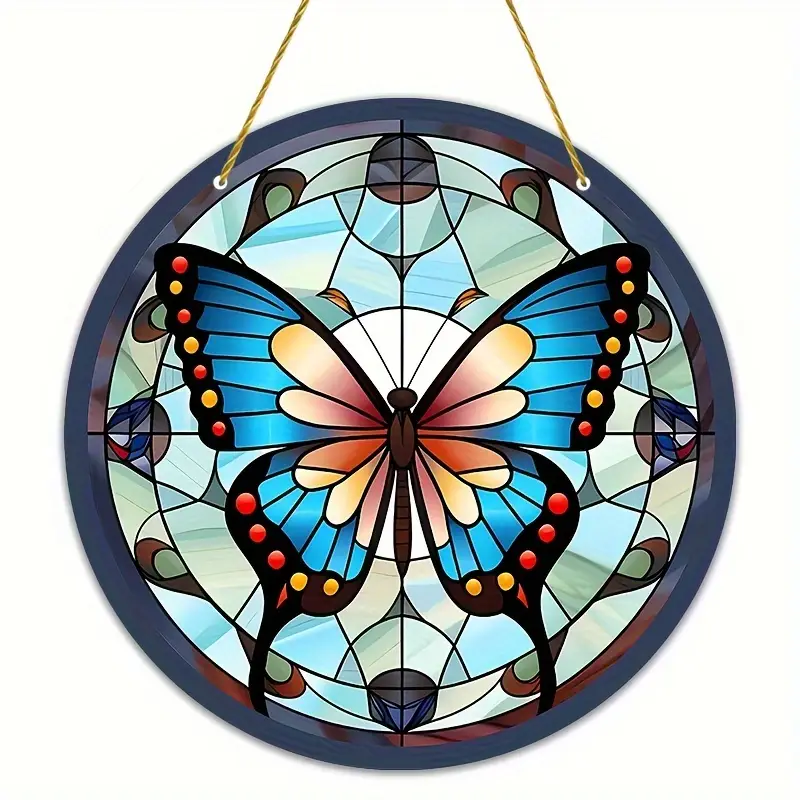The image depicts a circular stained glass window framed by a dark gray ring, hanging by two beige strings against a white background. Inside the window, a beautifully detailed butterfly takes center stage. The butterfly features a predominantly light blue hue, with distinctive black tips on its wings adorned with red and yellow dots. Its body is brown, and its wings exhibit a spectrum of colors, including yellow, orange, red, and hints of pinkish beige, with intricate blue accents near the edges. Surrounding the butterfly, the stained glass showcases a mosaic of pale green, blue, gray, and brown, creating an abstract and colorful backdrop. The overall composition, though complex in its color scheme, intricately combines these elements to form a vivid and elaborate stained glass artwork.